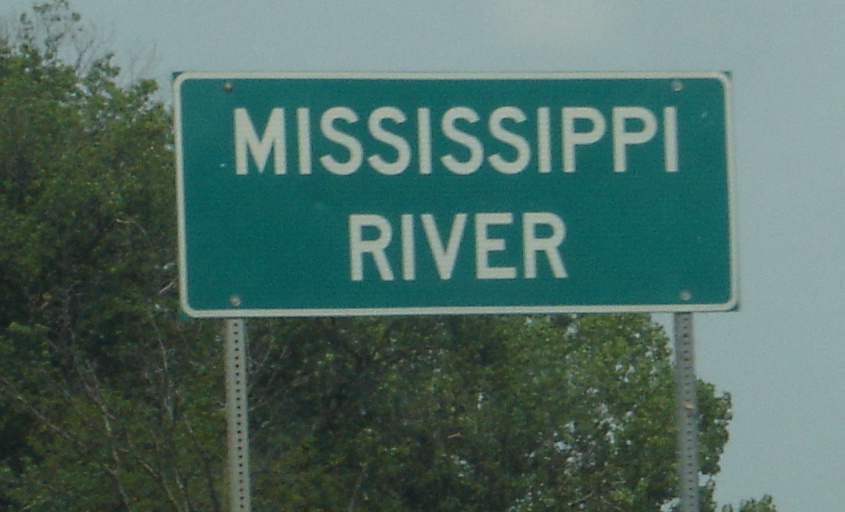This outdoor color photograph captures a road sign set against a partially overcast sky. The background features an expansive, pale blue sky covering the upper and right-hand sections of the image, while the left and lower portions are dominated by lush green foliage, perhaps a tree or a bush. The visual composition is almost evenly divided between the sky and the greenery, with the foliage slightly taking up more space. 

In the center of the frame stands a green road sign with a white border and bold, white lettering that reads "Mississippi" on the top line and "River" on the bottom line. The sign is supported by two gray metal posts that extend downwards and disappear out of the frame. The overall scene provides a straightforward yet picturesque view of this location marker amidst a natural, slightly cloudy setting.